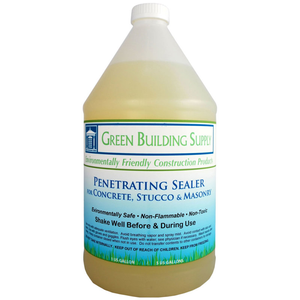The image depicts a white, semi-transparent plastic bottle with a cylindrical lower body and a conical upper section, topped with a small white screw cap. Inside the bottle, there is a yellowish liquid. The bottle features a label that starts white at the top and fades into blue at the bottom, with some text written in green, blue, and black. The label reads: "Green Building Supply," "environmentally friendly construction," and "penetrating sealer for concrete, stucco, and masonry." Additionally, it includes instructions such as "Shake well before and during use." The entire background of the image is white, emphasizing the details of the bottle and its label.